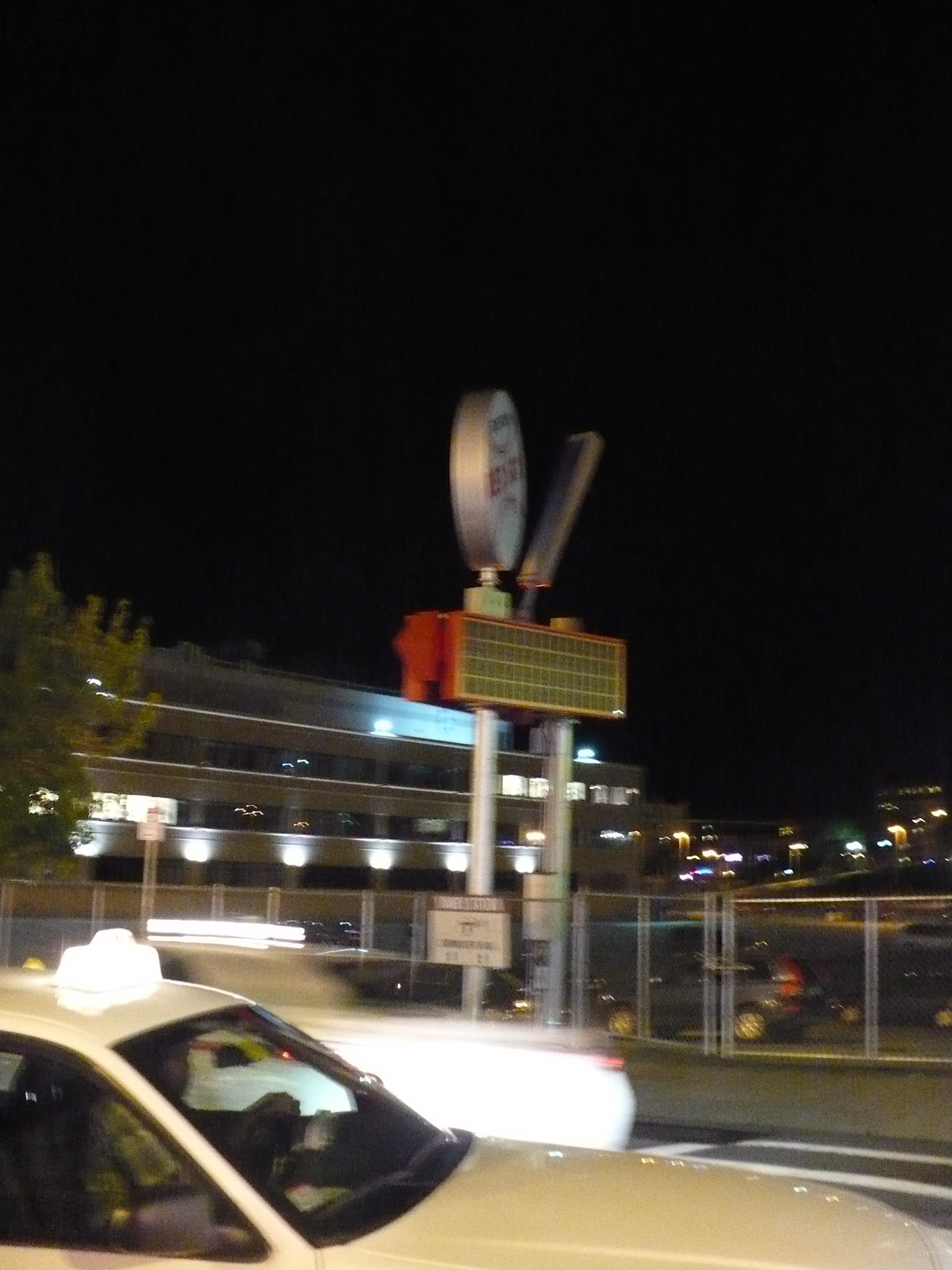This nighttime outdoor image, albeit low quality and motion-blurred, captures a scene under a pitch-black sky. Dominating the foreground is a white car moving towards the right, with a visible driver and a bright white light illuminating the top. Following closely behind, another car can be discerned, though its color remains indistinct due to the blur. In the background, a large sign stands prominently, central to the composition despite the image's graininess and low resolution.